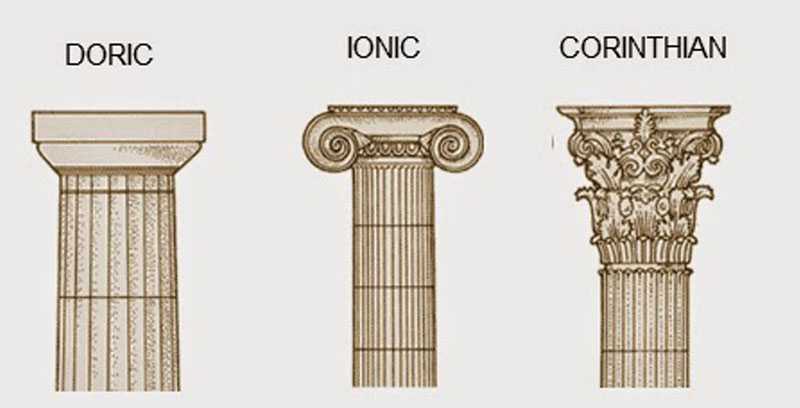This is a landscape layout image showcasing detailed black and cream drawings of three classical column types. Each of the three columns is identified with bold, all-caps labels above them. The left column is labeled "Doric," marked by a simple design featuring a rectangular capital that narrows down with horizontal grooves. The middle column, labeled "Ionic," has similar thin horizontal grooves, but its capital is distinguished by spiraling ram's horn-like volutes. The right column is labeled "Corinthian" and is the most ornate, with intricate floral and leaf motifs adorning its capital. These column styles, reminiscent of ancient Greek and Roman architecture, are displayed in distinct columns that reach the top of the image but are cut off at the bottom.